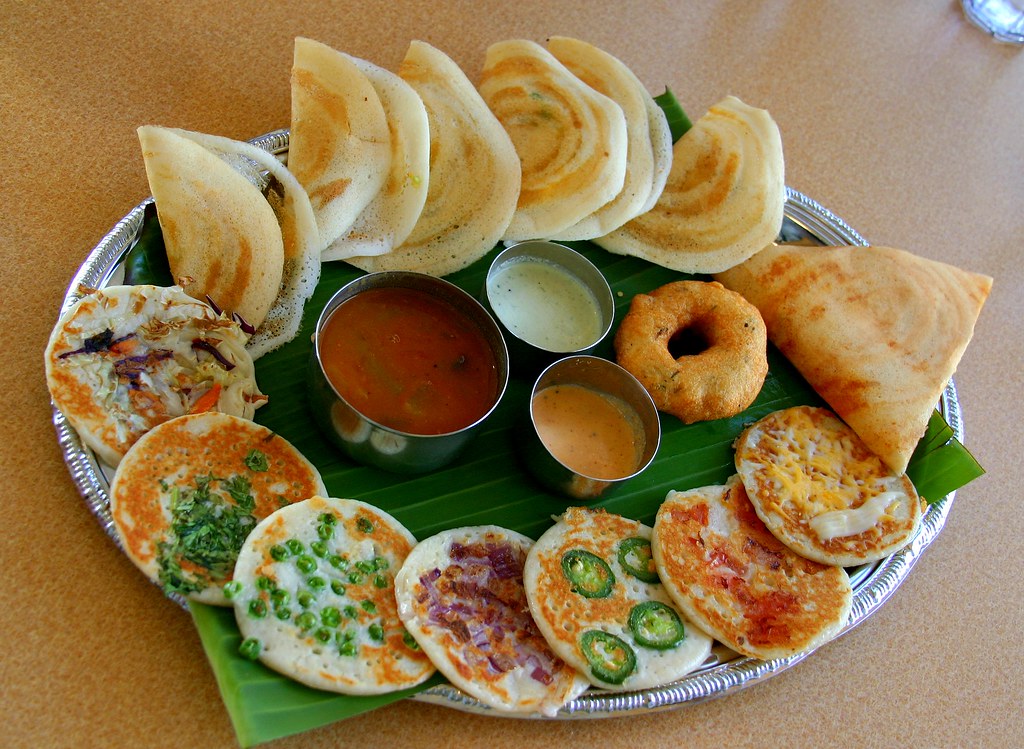The image displays an assortment of food items elegantly arranged on a silver platter, underlined with a green banana leaf. At the top of the plate, there are flexible, doughy dumplings that are slightly toasted on the sides and have a slightly oily sheen. One of the dumplings reveals a glimpse of its savory filling while the contents of the others remain concealed.

To the right, there is a wedge-shaped piece of bread, accompanied by a brown donut-shaped object. Three round metal containers are positioned strategically on the plate, each holding a different variety of sauce: one with a rich red sauce, another with a creamy white sauce, and the third with a vibrant pink sauce.

Additionally, there is a pancake-like piece of bread, white and toasted on the edges. These are generously topped with a variety of savory ingredients, including green onions, a mix of cheeses (American and Monterey Jack), red onions, and jalapeño peppers. The meticulous arrangement and diverse ingredients create a visually appealing and inviting setting.